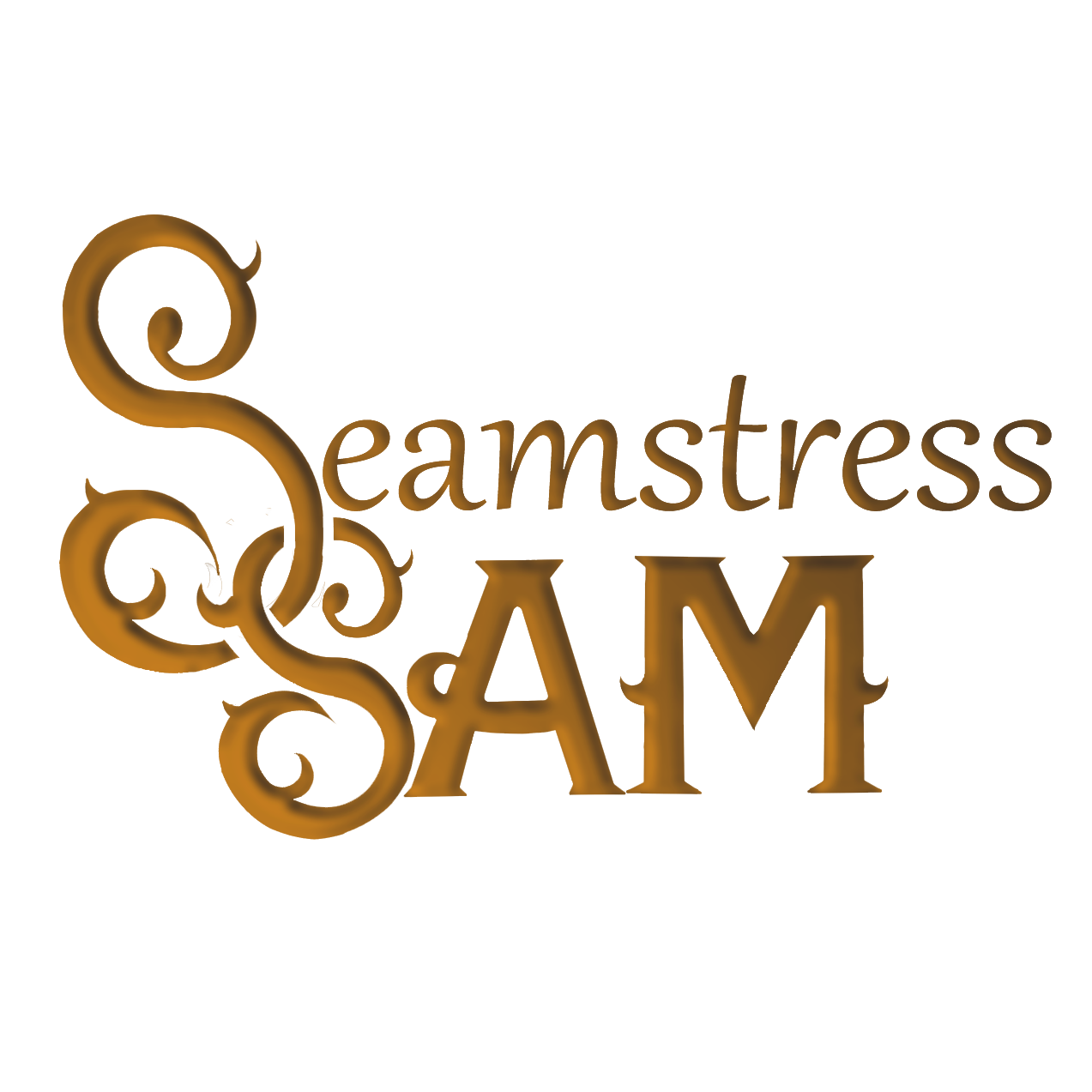The image features a business logo set against a solid white background, giving the impression that the logo is floating in an empty white void. The logo consists of two words, "Seamstress" on the top line and "Sam" directly below it, both rendered in the same light brown color. The text is centered in the image. The font used is fancy and detailed, with particular emphasis on the S's. The initial S in "Seamstress" and the S in "Sam" are intricately designed to look like thorn-covered vines. The top of the S in "Sam" wraps around the bottom of the S in "Seamstress," creating an interconnected visual effect. Additionally, the A in "Sam" has a thorn on the left crossbar, and the M features a small thorn on each side. The logo appears to be a scan or digital rendering and could likely represent branding for a company, suitable for business cards or letterheads.